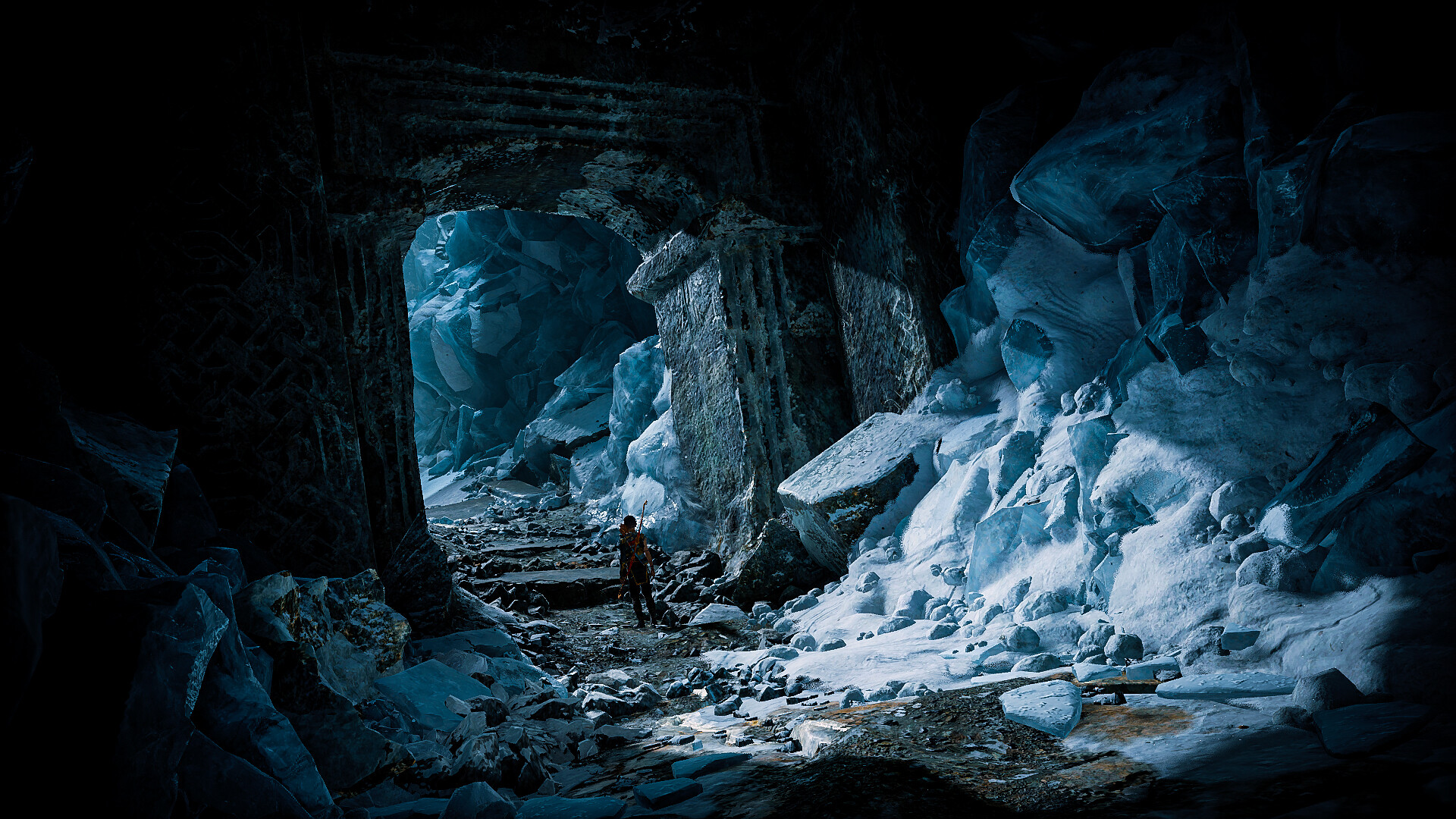This is a highly detailed color photograph or CGI image resembling a scene from a video game or animated series. Set inside a massive, ancient stone cave, the composition features a humongous archway dominating the center of the scene. Within this archway stands a minuscule human figure, cloaked in clothing including discernable pants and a shirt. The figure, though tiny compared to the towering cave, takes up roughly 5% of the frame, emphasizing the vast scale of the cavernous surroundings. 

Sunlight pierces through the archway from the left side of the image, casting a radiant beam that illuminates patches of pristine snow, creating a stark contrast against the otherwise bluish, dim, and ancient interior. This snow is piled both inside and outside the cave, with large boulders scattered throughout, suggesting the cave has remained untouched and unexplored for an extended period.

The overall scene has a dark and gloomy atmosphere, despite the sunlight highlighting the snow, which adds a touch of brightness to the otherwise subdued palette. The character appears to be exiting or entering this mysterious and expansive stone cavern, adding a sense of adventure and exploration to the scene.